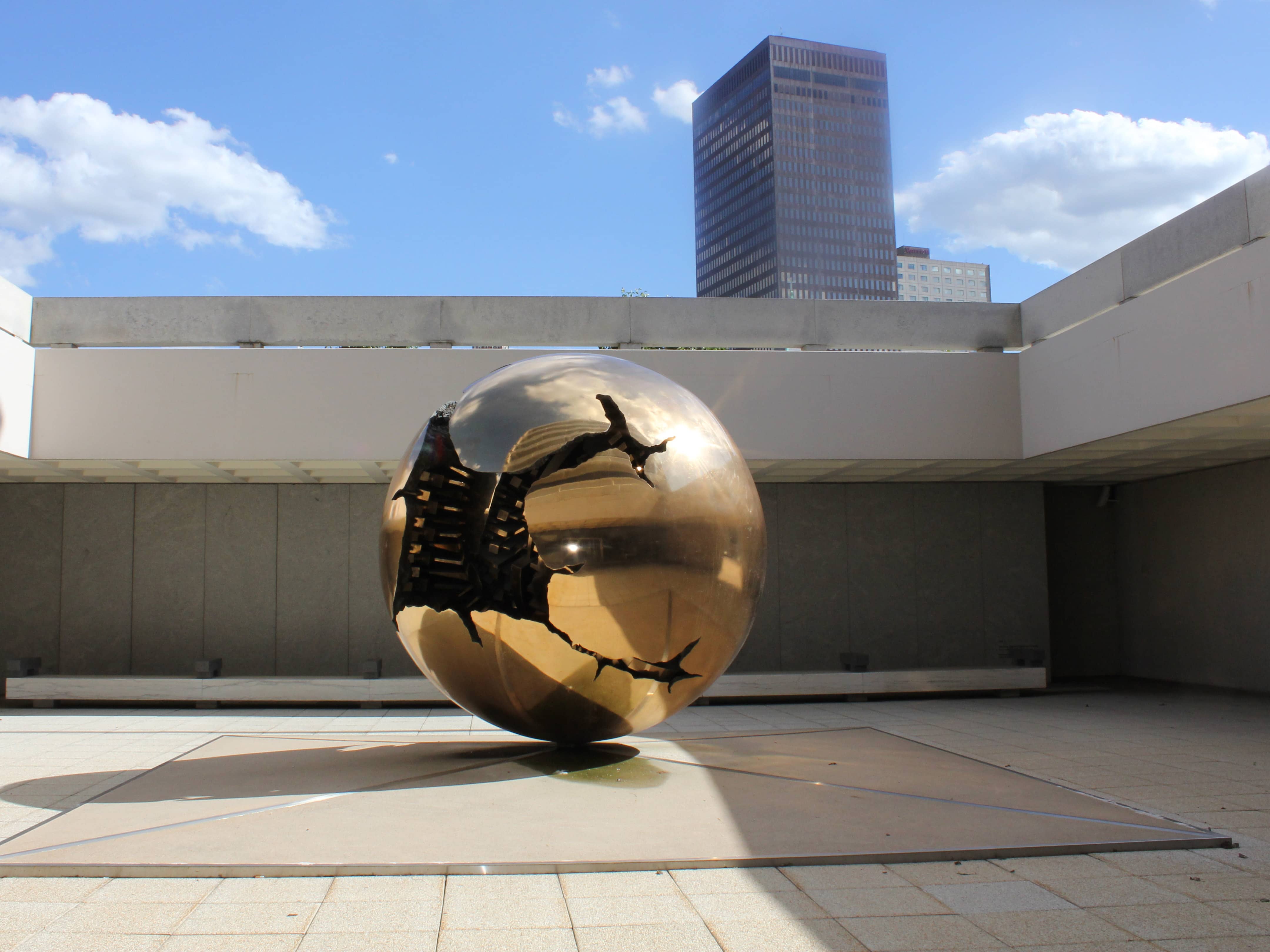This photograph, taken outdoors during the daytime, captures a striking art installation identified as the "Des Moines Art Display Sphere within a Sphere". At the center of the image lies a prominent, highly reflective silver sphere, which is slightly elevated on a pyramid-like concrete slab. The sphere features a large crack that offers a peek into its interior, revealing intricate, possibly computery parts, hinting at a possible alien or futuristic theme. The surrounding environment includes a larger concrete walkway, bordered by low concrete walls, leading to an open area under a blue sky dotted with large, fluffy white clouds. In the distance, tall skyscrapers punctuate the cityscape, adding an urban backdrop to this captivating scene. No people or benches are visible in the photo, which emphasizes the solitary yet eye-catching nature of the sculpture.